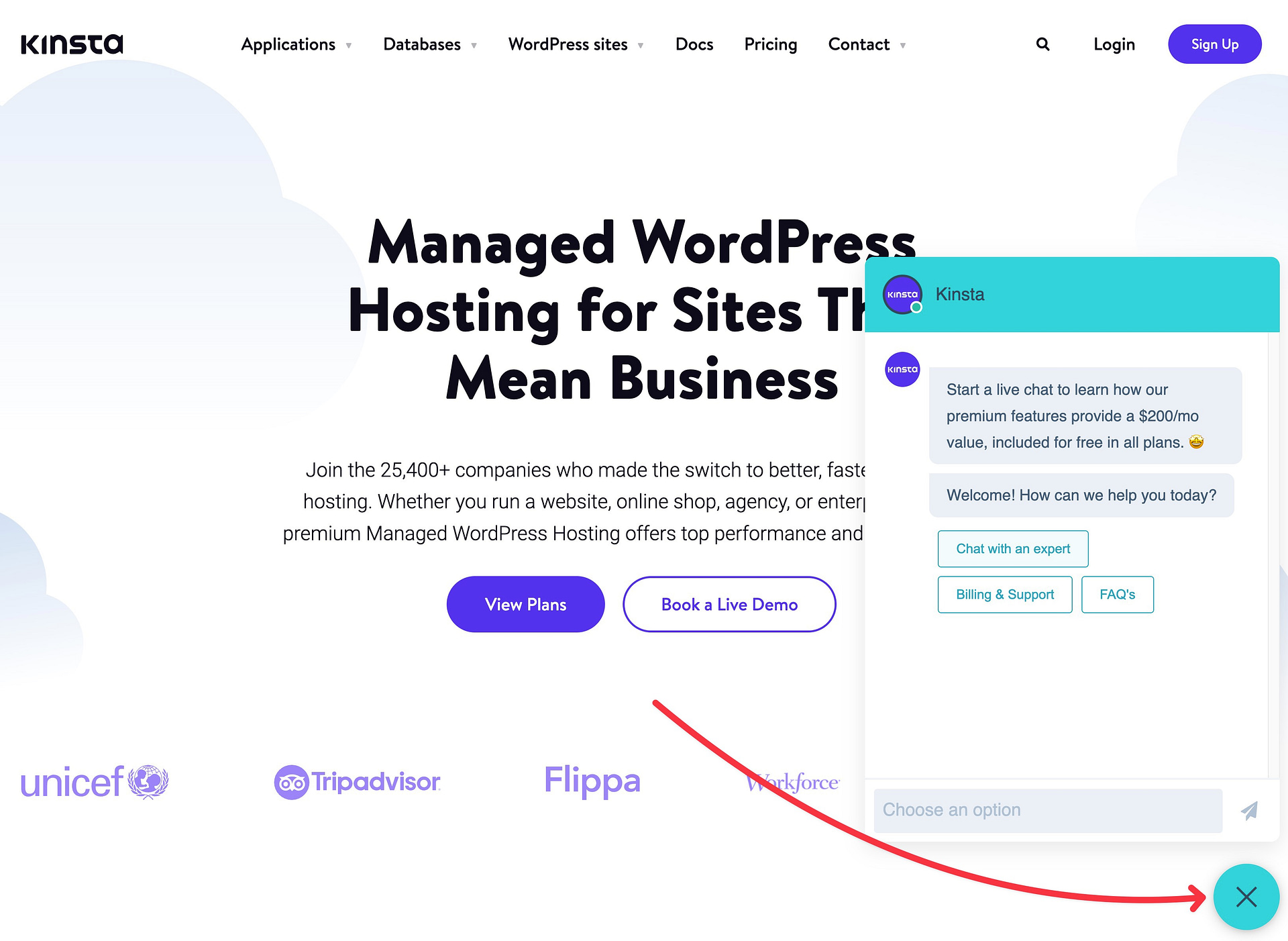This image displays a screenshot of the Kinsta website. At the top, prominently centered, is the bolded company name "Kinsta." To the right of the logo, and almost centrally located, are navigation links labeled "Applications," "Databases," and "WordPress Sites," each accompanied by a drop-down arrow. Following these links are additional options: "Docs," "Pricing," and "Contact," with "Contact" also featuring a drop-down arrow. On the right-hand side, there is a magnifying glass icon adjacent to the "Login" text, and next to it, a dark blue "Sign Up" button.

Centered in the middle of the page is a headline that reads, "Managed WordPress Hosting For Sites That Mean Business," although part of the text appears slightly obscured due to an overlay. Below this headline, a brief paragraph of descriptive text is visible, followed by two buttons: a solid purple button labeled "View Plans" and a transparent button labeled "Book a Live Demo." Additionally, a red arrow points to an "X" circle at the bottom.

An overlay message box is centered on the screen. It displays the company name at the top and includes a profile icon with a green dot. The body of the message invites users to "Start a live chat to learn how our premium features provide a $200/month value included for free in all plans," followed by further text, and features a selectable option area at the bottom for user interaction.